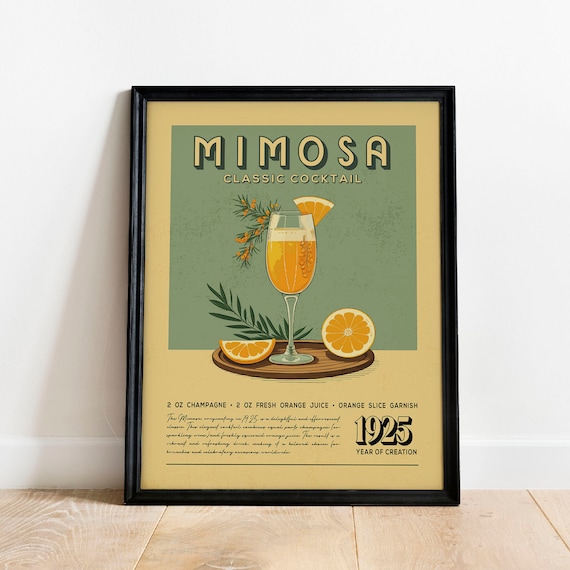The image is a horizontally rectangular framed poster, leaning against a white wall with a slight bottom extension, and sitting on a polished wood floor with visible planks. The black narrow wood frame encloses the poster's yellow background which features a light blue square in the top half. In this square, the word "Mimosa" appears in all capital letters with a shadow effect, accompanied by the subtitle "Classic Cocktails." Below, there is a brown tray showcasing a bubbly mimosa in a glass, garnished with an orange zest and a sprig of leaves. The tray also holds a half-sliced orange and an additional orange slice resting on its back. At the bottom of the poster, in fine print too small to read, are likely the mixing instructions for making a mimosa. The year "1925" is clearly displayed in the lower right-hand corner, indicating the mimosa's year of creation.